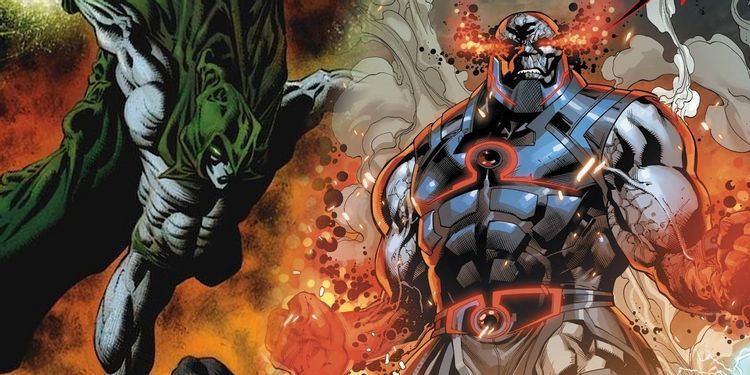The image appears to be a dynamic scene from a comic book featuring two intensely muscular superpowered beings, likely superheroes or perhaps supervillains, locked in a fierce battle or poised to team up in destruction. In the background, fire, explosions, and billowing smoke hint at a landscape ravaged by their immense power.

On the left, a massive figure described as a gray-skinned man with an extremely muscular physique, practically boasting an exaggerated number of abdominal muscles, is in mid-flight. He wears a flowing green cape and hood, and possibly green shorts, though shadows obscure much of his lower body. His face is adorned with distinctive makeup or markings, further emphasizing his rage. His wide jaw, clenched teeth, and venomous expression make him look menacing as he descends, fists at the ready.

To the right is another imposing figure, equally muscular, clad in blue armor with glowing red accents. His suit extends over his abs, creating a formidable chest plate that highlights his immense strength. This character's eyes and fists blaze with fire, and smoke whirls around him, suggesting he possesses powerful, flame-based abilities. His posture is aggressive, with clenched fists and fire shooting from his eyes and hands, projecting an aura of raw, uncontrolled power.

Together, these two powerful beings create a vividly intense and colorful graphic depiction, whether allies or adversaries, embodying the high drama and explosive energy characteristic of intense comic book action scenes.